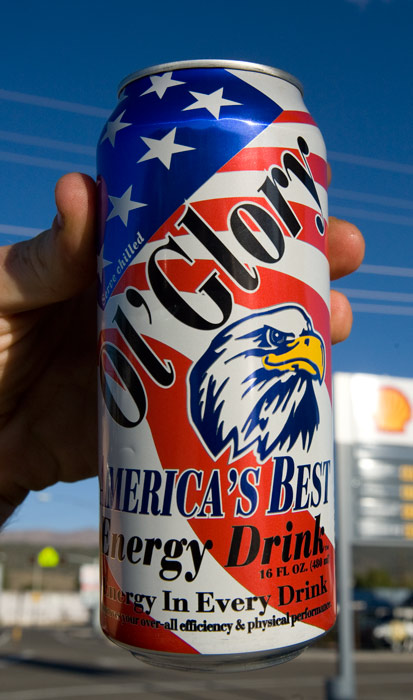A detailed caption for the image can be:

"In this vibrant photograph, a hand is prominently holding a can of energy drink adorned with an American flag and a striking illustration of an eagle's head facing the right. Bold letters on the can read 'All Glory,' emphasizing its patriotic theme. Additional text on the can promotes it as 'America's best energy drink,' boasting a volume of 16 fl oz and promising 'energy in every drink' with claims of 'overall efficiency and physical performance.' The background features a blurry Shell gas station sign and what appears to be a trailer for a semi-truck, adding context to the location. Above, a clear blue sky crisscrossed with power lines completes the scene, highlighting the juxtaposition of everyday American life with the patriotic branding of the energy drink."